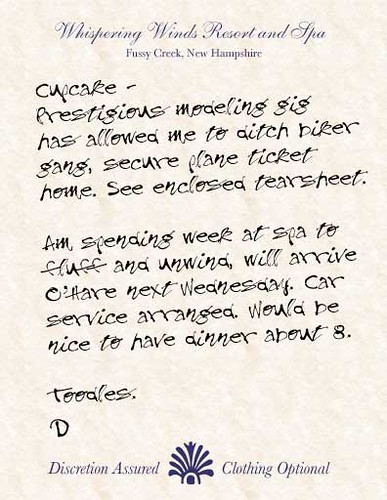The image shows a cream-colored piece of stationery from Whispering Winds Resort and Spa in Fussy Creek, New Hampshire. At the top middle of the stationery, the name of the resort is elegantly printed in a lilac-colored font. Below this, a handwritten note in black ink addresses 'Cupcake.' The note reads: "Cupcake, Prestigious modeling gig has allowed me to ditch biker gang, secure plane ticket home. See enclosed tear sheet. Am spending week at spa to fluff and unwind. Will arrive here next Wednesday. Car service arranged. Would be nice to have dinner about 8. Toodles, D." At the bottom middle, there's a logo flanked by the phrases "Discretion Assured" on the left and "Clothing Optional" on the right. The overall feel of the stationery and the note reflects a sophisticated and exclusive resort experience.